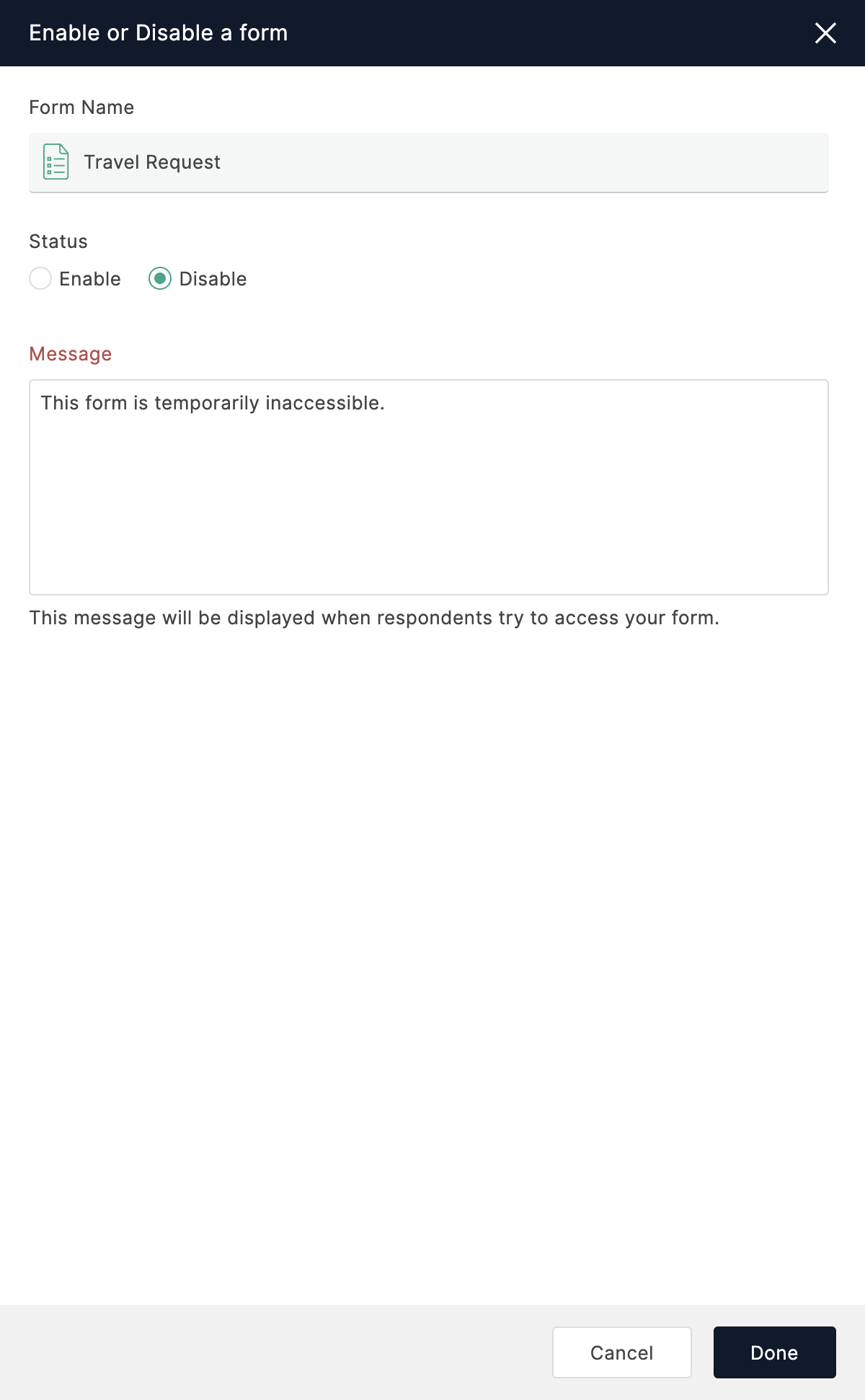The screenshot showcases a user interface for enabling or disabling a form. At the top, a black status bar spans the width of the screen, featuring white text that reads "Enable or Disable a Form." On the far right of this bar, there is an 'X' icon for closing the window.

Below the status bar is the "Form Name" section. An aqua-colored icon resembling a memo with a slightly turned-up corner is present, and to its right is the form’s name, "Travel Request," displayed in darker gray text. 

Under the form name, a "Status" section is visible, featuring two side-by-side toggle buttons labeled "Enable" and "Disable." The "Disable" option is currently selected, indicated by its slightly darker color.

Further down, there is an orange message indicating that modifications are in progress. The subsequent section is titled "Message," followed by a large message input box in which the black text states, "This form is temporarily inaccessible." This message is repeated within the input box. Below it, another line of black text clarifies that "This message will be displayed when respondents try to access your form."

To the bottom right of the screen, ample white space precedes two buttons: a white "Cancel" button with black text and a black "Done" button with white text.